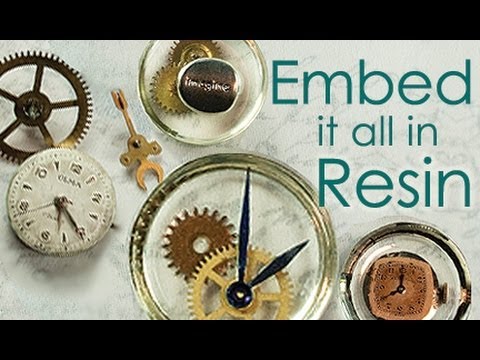The image features a detailed arrangement of watch parts and clock faces, prominently set against a background with a whitish greenish marble tint. At the very top and the bottom of the image are bands of black. On the right side, text in green reads "embed it all in resin." Below this text is a clear glass bowl with a gold rim, containing a round, resin-embedded clock with both minute and hour hands. Adjacent to this bowl is another clear bowl with a similar gold rim, holding what appears to be a polymer clay clock featuring two round wheels and clock hands. 

There is also a wider, gold-colored ring with a central gold gear and a smaller, rusted brown gear. Above these elements is another gold gear. Off to the side is a small, square watch face with black hands, accompanied by another larger clock face that is white with numerals and markings from 12 to 2, and includes an hour, minute, and second hand. Additionally, there are clock parts with round wheels and gears scattered throughout the composition. A distinct gold-rimmed circle at the top bears the word "imagine," tying together the artistic and functional elements of clock mechanisms showcased in a resin embedding tutorial.